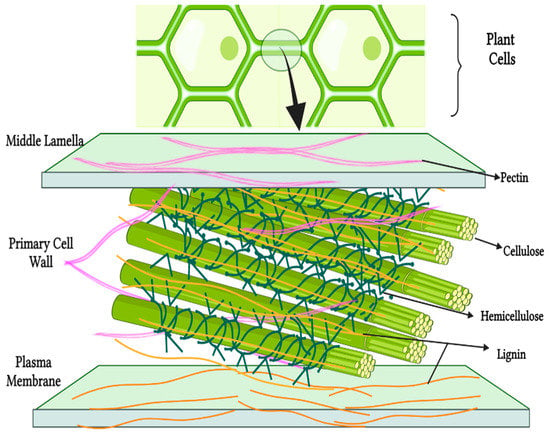This is an illustrated image set against a white background, featuring labeled diagrams of plant cell structures. At the very top, the image shows interconnected green hexagons encircled with an arrow pointing downward, labeled "plant cells." Below this, there's a teal-colored, rectangular sheet placed on its side, labeled "middle lamella," with purple veins and a black line indicating "pectin." Directly beneath the middle lamella, several cylindrical, green stalks are bundled together like sticks, marked with arrows identifying "cellulose," "hemicellulose," and "lignin." To the left of these stalks, the image is labeled "primary cell wall." Additionally, the middle part where the cylindrical objects are bundled shows the "lignin" pointing to orangish parts, and "hemicellulose" pointing to darker green twirling vines. At the bottom, another teal rectangular plane with orange veins, labeled "plasma membrane," sandwiches the primary cell wall structures.